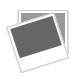The image features a weathered, cracked wooden fence, visible primarily in the lower left corner and extending up the left side and a bit at the top. Mounted on the fence is a poster showcasing a collection of aged, worn science fiction paperbacks. The books are arranged in seven overlapping rows, each book partially covering the one beneath it. The titles on the top row include "E.E. Doc Smith," "Arthur C. Clarke's Venus Prime," and "faster than a computer deadlier than a laser the big brain," followed by "hero." The collection, which appears to be approximately 28 books in total, includes illustrations of astronauts and planets, suggesting a strong sci-fi theme. The display rests on a white tablecloth over an old wooden table.